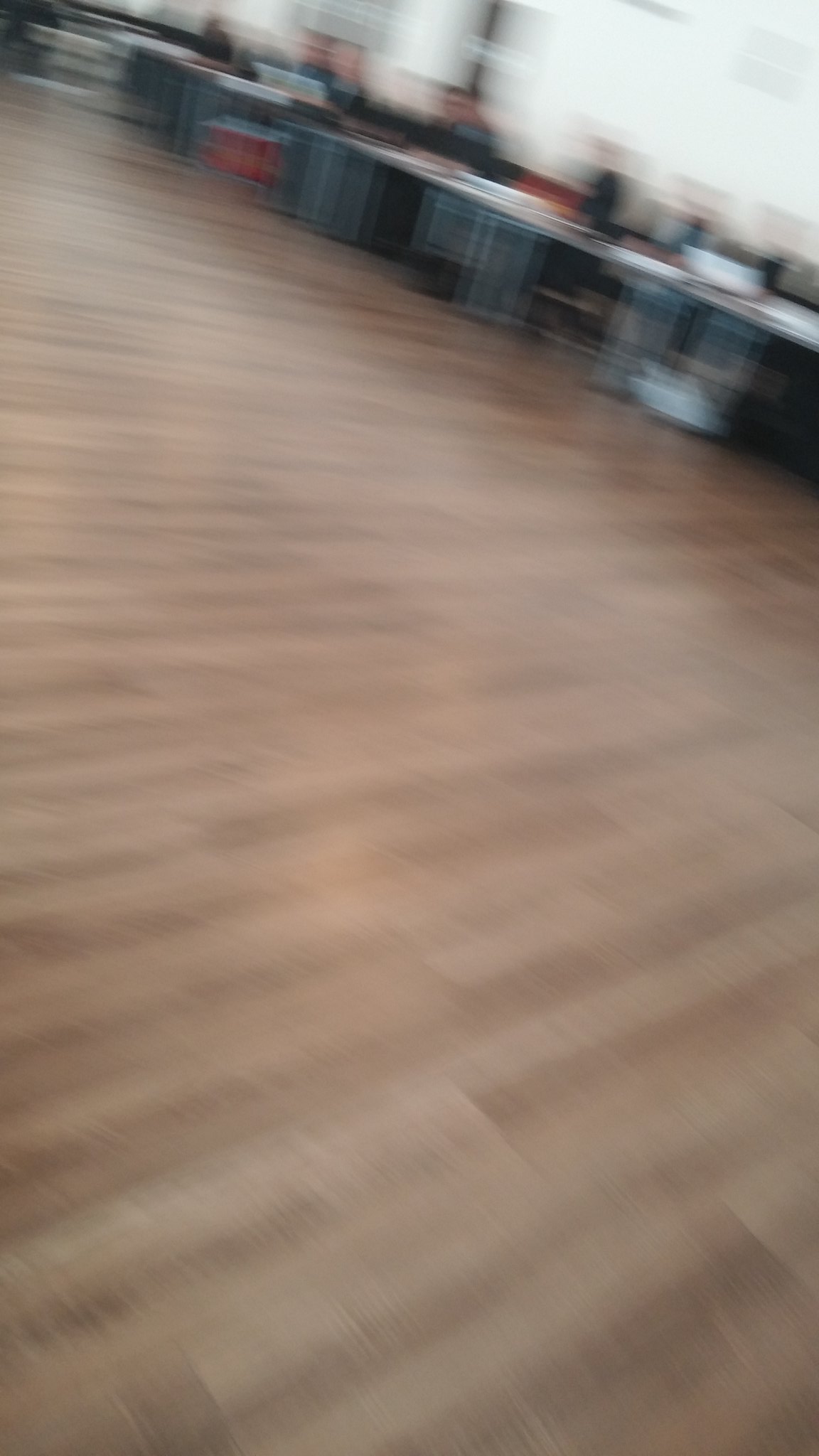In this blurry photograph, although the primary focus seems to be on a wooden floor, the backdrop appears to depict an office setting. The floor is made of hardwood, providing a rich, warm texture that extends throughout the image. Towards the background, albeit still hazy, several desks can be discerned. In the upper left-hand corner, a red cooler is faintly visible, contributing a pop of color to the otherwise muted scene. Additionally, approximately two or possibly three individuals are seated at their desks, though the blur makes it challenging to confirm exact details. The back wall of the office is painted white, creating a crisp contrast to the floor. The entire image is slightly tilted to the right, adding an unintended dynamic element to the composition. There is no text overlay, ensuring the viewer's attention remains on the visual elements.